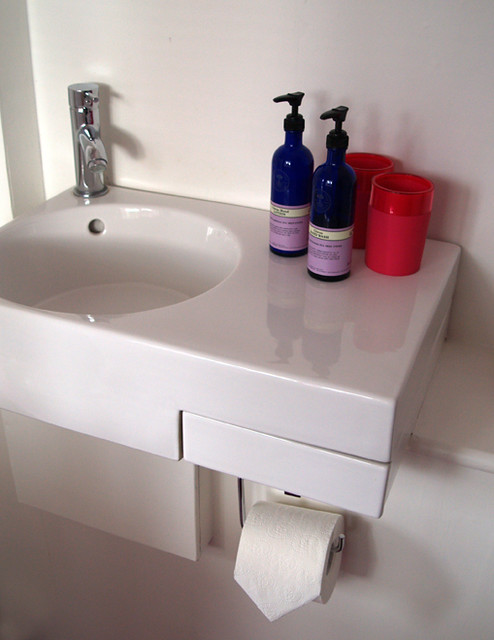This photograph features a meticulously arranged bathroom sink, likely situated in a hotel room. The centerpiece is a round, ceramic porcelain sink with an integrated metallic faucet and control fixture. To the left of the sink, there is a small countertop area holding two vibrant red glasses and two large blue bottles of lotion, both equipped with plunger tops. On the right side, a drawer is present beneath the sink, and just below it, a roll of toilet paper has been thoughtfully prepared with a pointed end—an attention to detail often seen in hotels to signify cleanliness and readiness for new guests. The entire area, from the glistening sink to the neatly arranged toiletries, exudes a sense of meticulous care, ensuring a welcoming and hygienic environment for the next occupant.